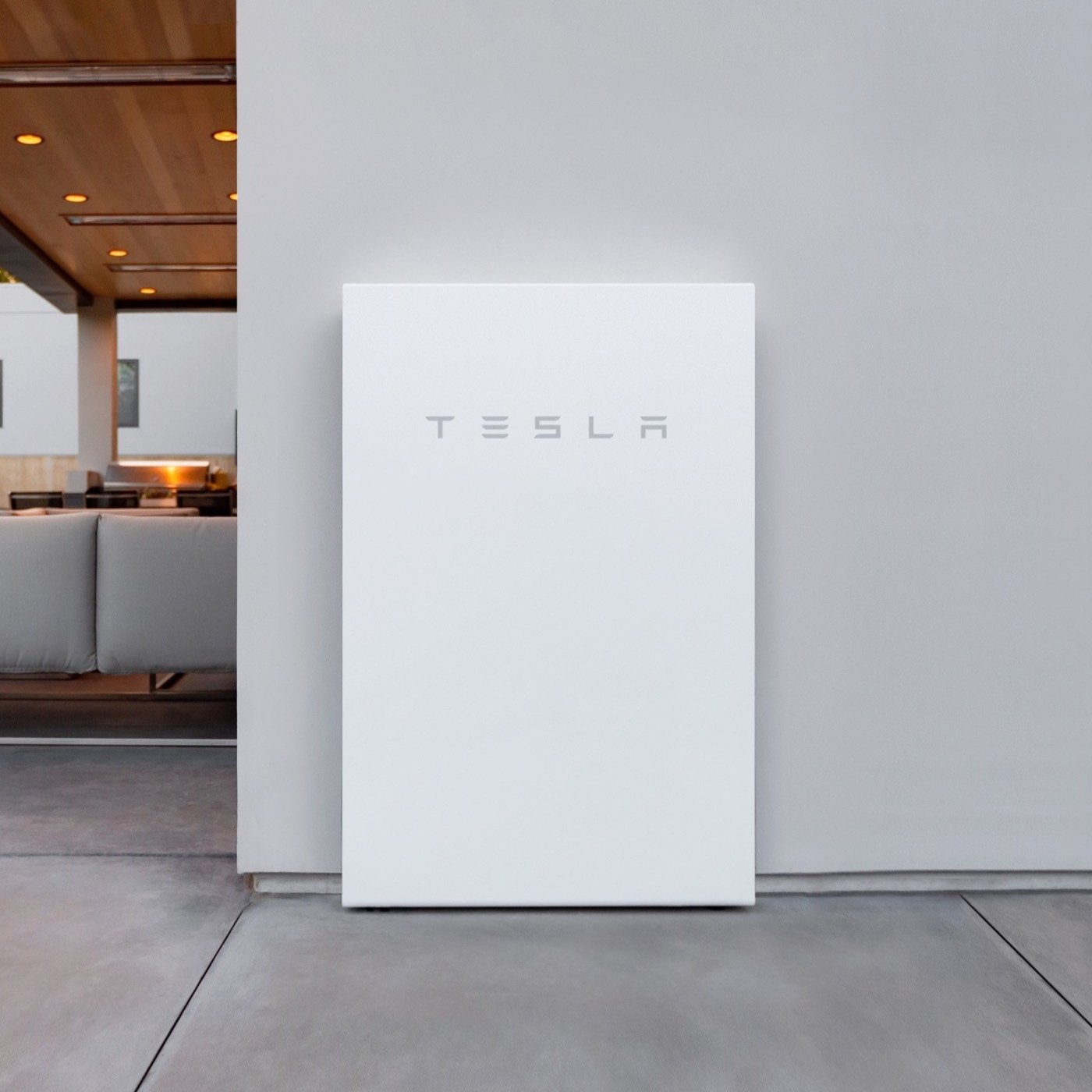The image is a color photograph showcasing the interior of a modern building. The left side of the frame is occupied by the back of gray couches, aligning with a sleek, wood-paneled ceiling adorned with recessed can lights. The floor appears to be made of smooth, poured concrete, adding to the contemporary aesthetic of the space. Centered in the composition, a gray wall serves as a backdrop for a large, white rectangular object propped against it. This object prominently features the distinctive gray Tesla logo across its front, and it rests on the same concrete floor, blending seamlessly with the overall minimalist design.